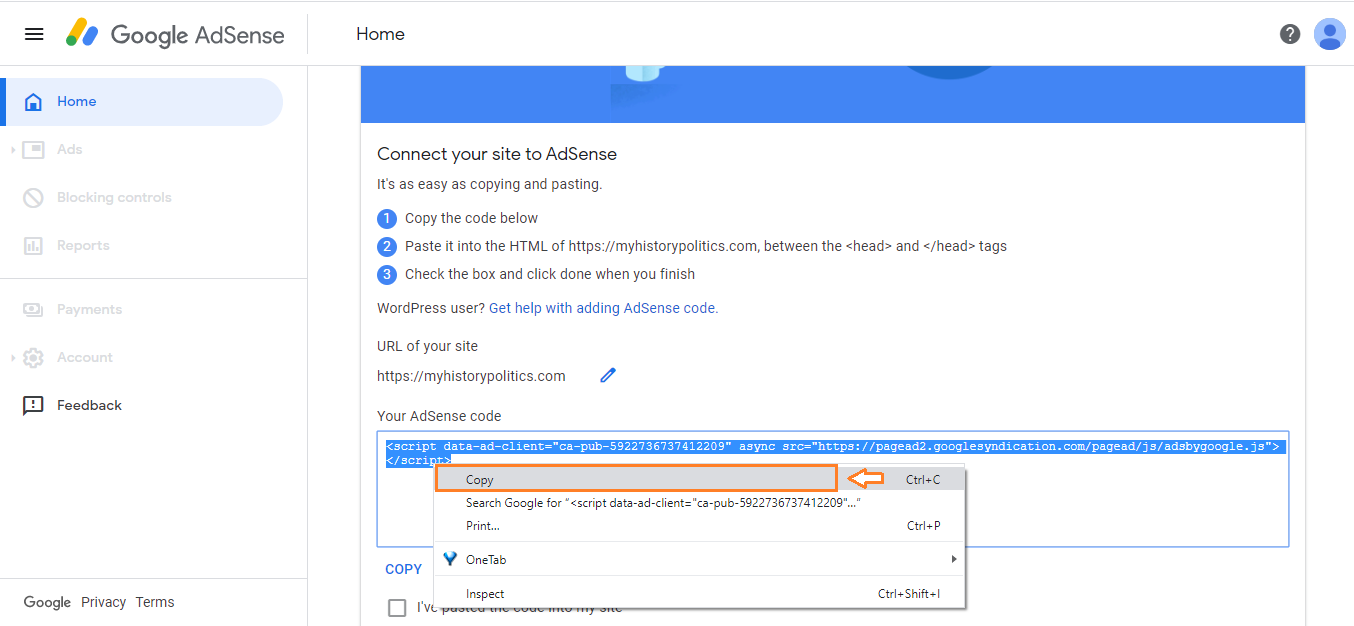In this screenshot of the Google AdSense homepage, the interface is divided into distinct sections. On the left-hand side, a navigation menu lists options including Home, Ads, Blocking Controls, Reports, Payments, Account, and Feedback. The central portion of the screen prominently features a message encouraging the user to connect their site to AdSense, highlighting the simplicity of the process. It instructs users to copy a provided code and paste it into the HTML of their website, MyHistoryPolitics.com, specifically between the `<head>` tags. For WordPress users, a convenient link is provided to facilitate this step. An arrow points towards the AdSense code, marked by a pin, signaling where to click to copy the code. At the bottom, there's a mention of the Google Privacy Policy in clickable blue text.